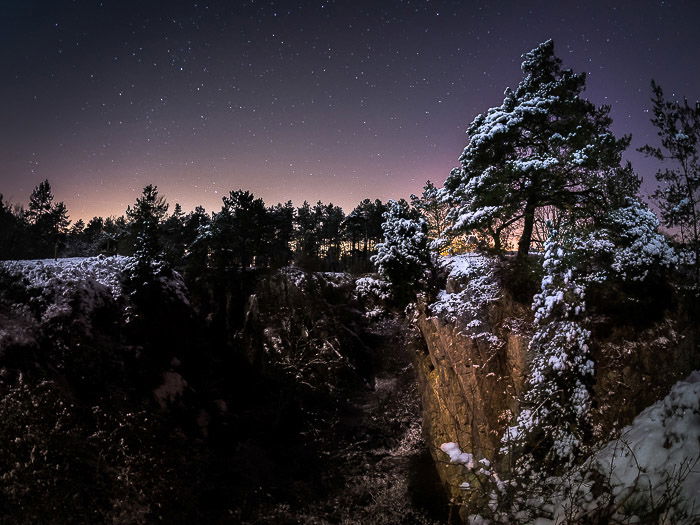A stunning night photograph captures a cliffside ravine during winter. The snow-covered ground and trees contribute to the serene, frosty ambiance. The sky, occupying the upper third of the image, transitions from a deep dusky purple to a lighter violet-pink closer to the horizon, which is adorned with a tree line. Stars speckle the sky, enhancing the night-time atmosphere. The ravine, stretching horizontally across the image, dips into a U-shape at its center. Along the edges of the cliff, trees stand adorned with snow, including one prominent triangular pine tree on the right, heavily laden with snow, perched on a particularly jagged, brown section of the cliffside that contrasts with the predominantly black and white landscape. A fallen tree, also covered in snow, hangs off the edge, adding to the rugged wilderness of the scene. At the bottom of the ravine, dark tan rocks suggest the presence of a creek or stream running through it, completing this tranquil and picturesque winter tableau.